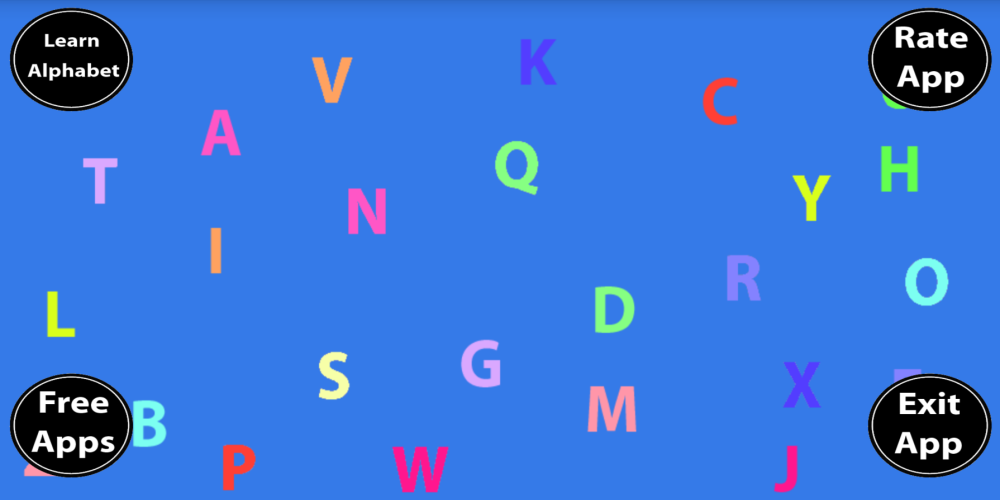The image showcases a horizontally elongated, blue rectangle with four black circles, each placed in one of the corners. The circles contain white text and serve as buttons with the following labels: "Learn Alphabet" in the upper left, "Rate App" in the upper right, "Free Apps" in the bottom left, and "Exit App" in the bottom right. The background is adorned with various colorful uppercase letters scattered throughout. These letters come in a myriad of hues, including shades of pink (light, dark, and medium), orange, green, blue, purple (light and dark), and yellow. The design and arrangement of the letters evoke the appearance of magnetic alphabet toys traditionally used by children for learning, suggesting an educational application aimed at teaching kids the alphabet. The vibrant and playful visual elements indicate a user-friendly and engaging interface for young learners.